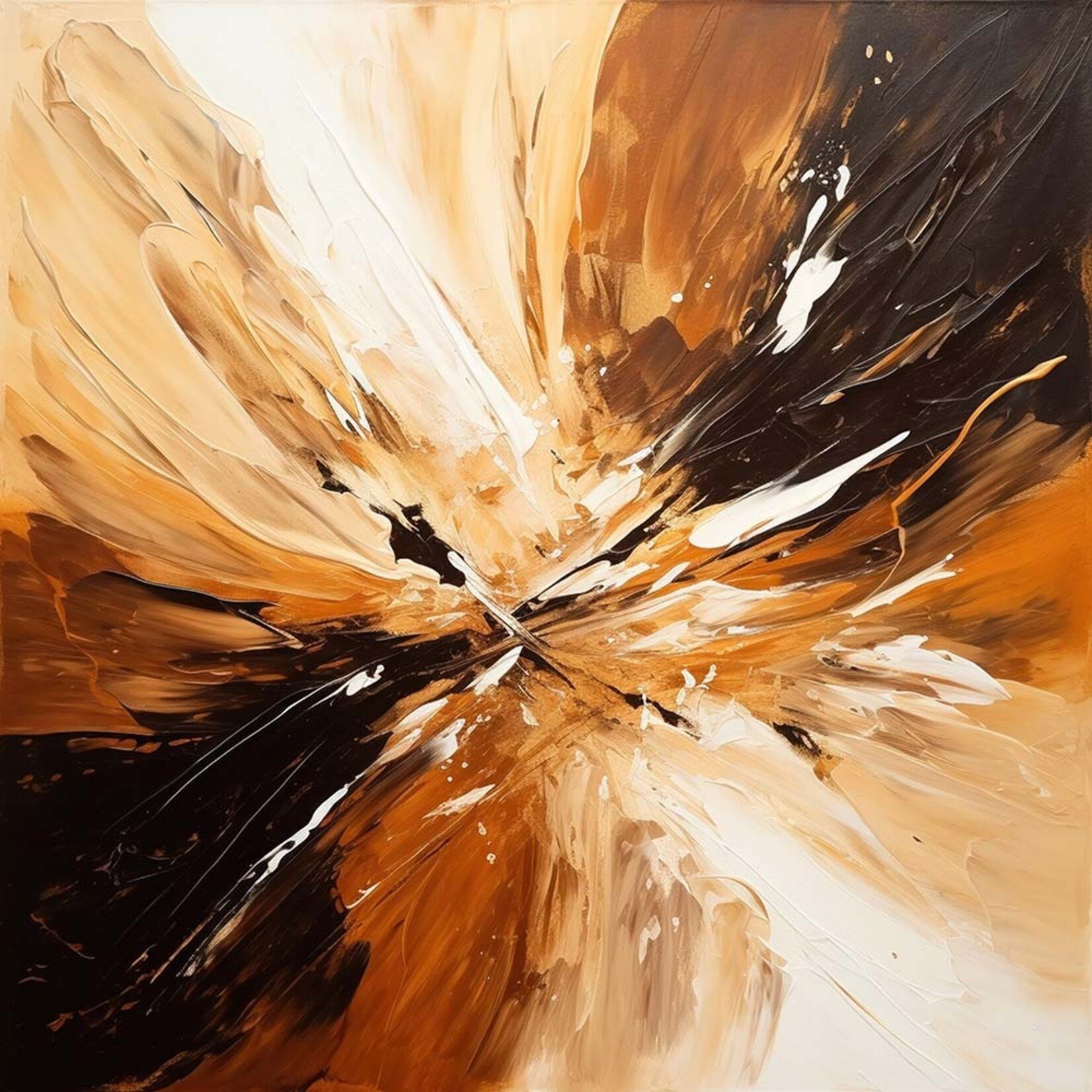This image is an abstract, modern painting, primarily composed of brown and tan hues with dramatic splashes of dark brown and white paint. The composition seems to radiate towards the center, creating a dynamic and visually striking effect that almost resembles flowing water or wind. The top left to bottom right and bottom left to top right corners feature splatters of dark brown, transitioning through shades of tan to light brown and white. The painting also includes visible brush strokes, adding texture and depth. Diagonally across the canvas, there are splashes of dark brown and black with white highlights, giving the impression of two shadowy figures rushing towards each other. The overall effect is very textured, full of movement, and visually intriguing, capturing the essence of abstract art with its layered and flowing elements.